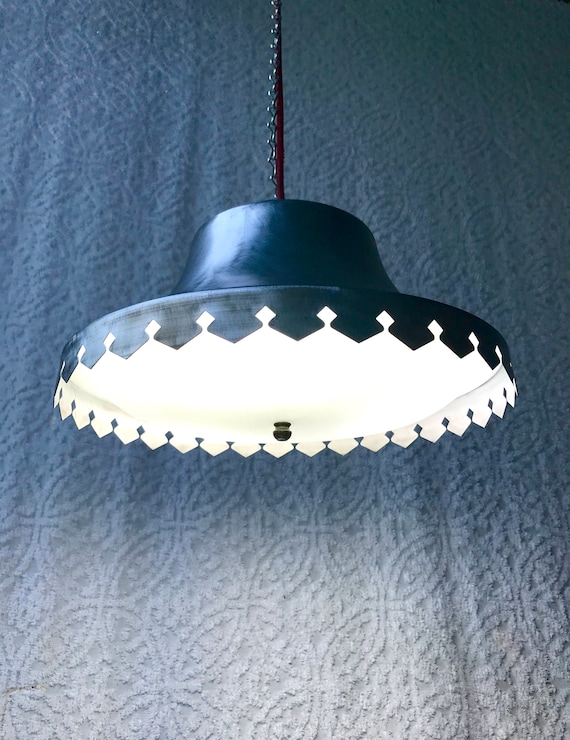A photograph captures an elegant, vintage chandelier, possibly dating back to the 1950s, hanging from a textured white or light blue curtain with a circular pattern. The chandelier is suspended by a braided cord and silver chain, giving it a classic diner aesthetic. The top portion of the chandelier is a dark blue, sombrero-shaped metal structure with an overhanging brim adorned with horizontal diamond-shaped cutouts. Between these cutouts, vertical white spaces form additional diamond patterns. The overall design converges into a pointed tip while the round glass centerpiece has a little brown knob for unscrewing. The light from the bulb illuminates underneath, creating a bright focal point in contrast to the darker upper part of the image.